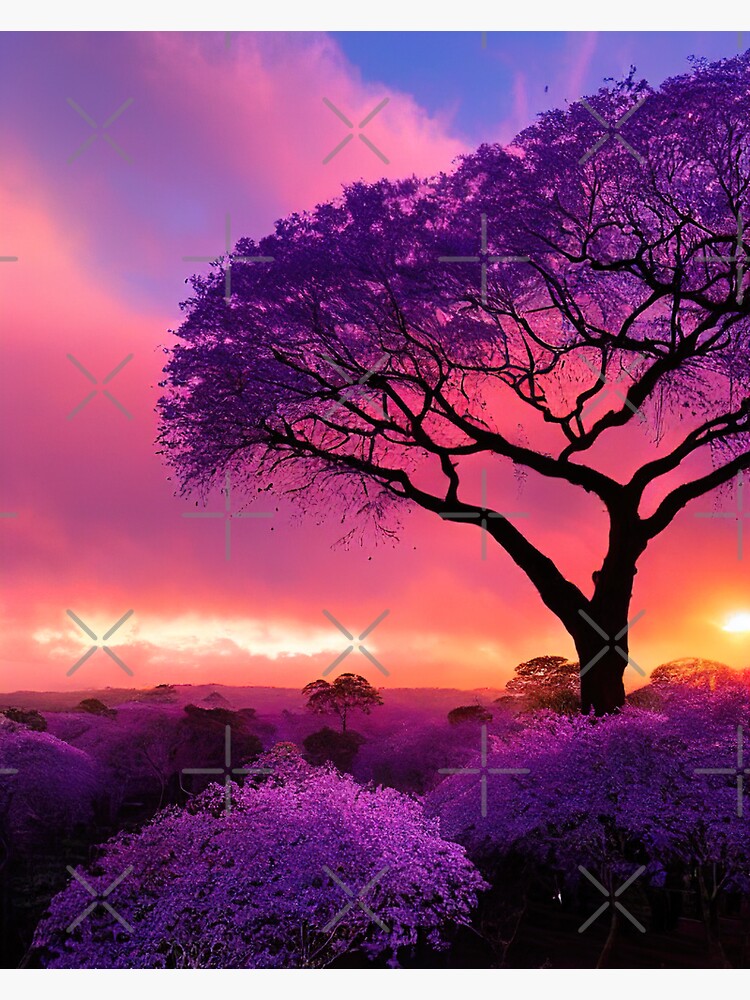In this surreal and vividly colored image, we are presented with a computer-generated depiction of a fantastical, African-like treetop landscape. Dominating the scene is a majestic tree of life, its trunk and multiple branches silhouetted in dark hues, extending prominently from the center towards the upper right corner. The tree stands above a sea of canopies, adorned with vibrant purple leaves that do not extend downward but cluster only at the top. These tree canopies fill the image from the center to the right edge, where some of the leaves are cut off. Beneath this treetop layer, the ground is punctuated by patches of dark purple shrubbery, giving an impression of depth and texture.

The sky above is a mesmerizing blend of purple, pink, orange, and yellow, with white and pink clouds breaking through to reveal glimpses of blue. This kaleidoscope of colors evokes the aura of a blazing sunset or sunrise. The landscape below is bathed in the surreal glow of these vivid hues, with a particular yellow line near the bottom center hinting at the sun peeking through. Adding to its otherworldly feel, the image is overlaid with broken Xs and crosses, as though viewed through a fragmented grid, enhancing its dreamlike, ethereal quality.